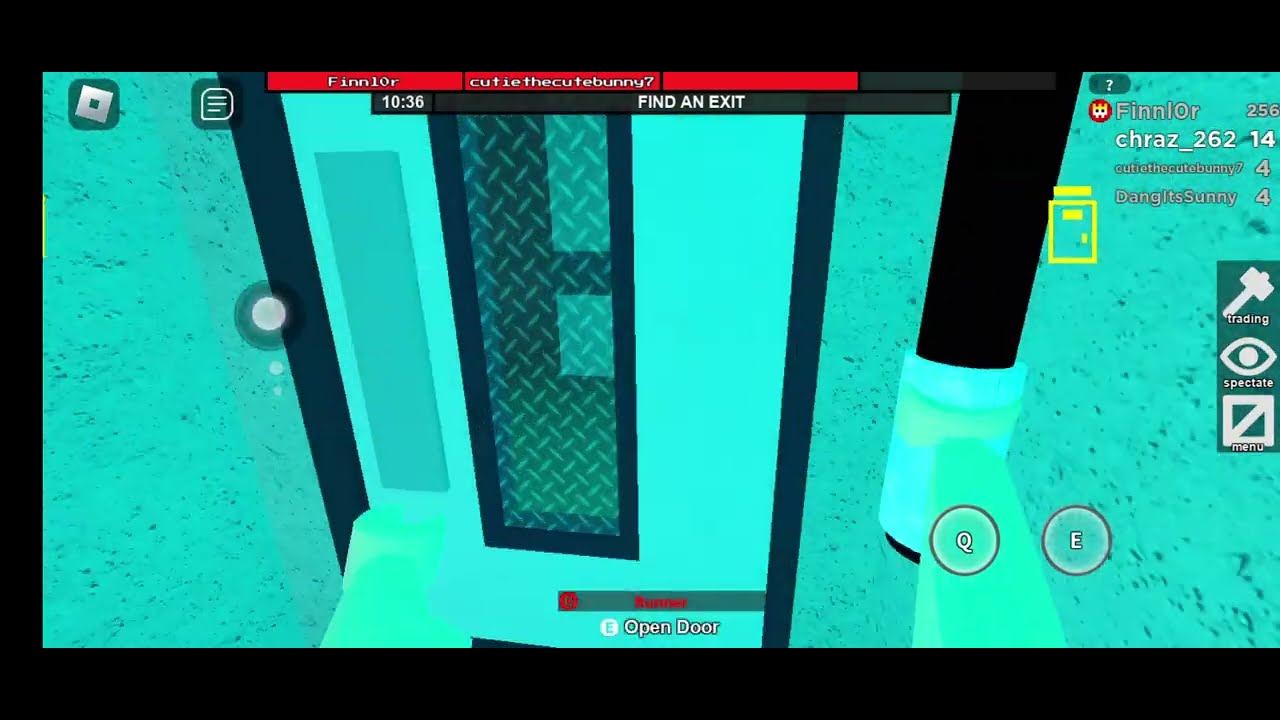The image is a rectangular screenshot from a video game featuring a predominantly blue, green, and black color scheme, giving it an underwater ambiance. The scene showcases a steel door with a rectangular window reinforced with metal wiring. The view is framed by a black header and footer and a black border on the left but not on the right. The top of the screen displays a red banner with player names "Finnear" and "Cutie, the Cute Bunny," along with a game directive, "Find an Exit," and a time stamp, "10:36." In the bottom area, there's a clickable link labeled "Open Door." The top right corner includes additional player information, notably "Finnear's" emblem and numbers "256" and "CHRAZ_26214," alongside other monikers and scores. Below this, icons for "Trading," "Spectate," and "Menu" options are visible with control keys "Q" and "E." The central focus reveals a yellow-outlined door with two hands reaching out towards it—one grasping a black bar and the other extended forward, emphasizing the gameplay's objective of navigating through different rooms to find an exit.